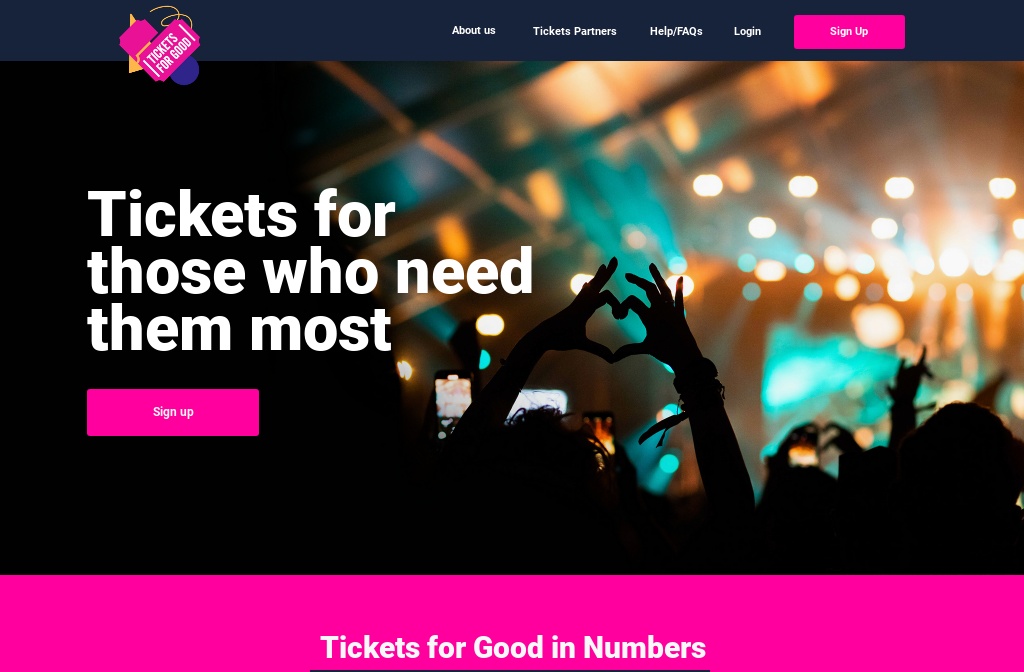The website features a distinct logo that reads "Tickets for Good," presented on a pink, vintage-style single ticket angled slightly to the side. The text appears on the ticket, which is overlaid upon a more silhouetted ticket, together forming a near heart shape. The background includes various miscellaneous shapes: a triangle, a semi-circle, and a spiral string.

At the top of the page, navigation options are clearly laid out: 'About Us,' 'Ticket Partners,' 'Help/FAQ,' 'Login,' and 'Sign Up.' A prominent white text slogan, "Tickets for Those Who Need Them Most," spans the majority of the screen, with a 'Sign Up' button positioned just below.

The main visual is an engaging scene from a rave or concert, showcasing the audience in silhouette. Several individuals are holding up phones, capturing videos of the stage. Central to this image is a person in the middle of the crowd, making a heart shape with their hands by touching their index fingers and thumbs together.

At the bottom of the webpage, a hot pink block prominently displays "Tickets for Good" followed by relevant numerical statistics.